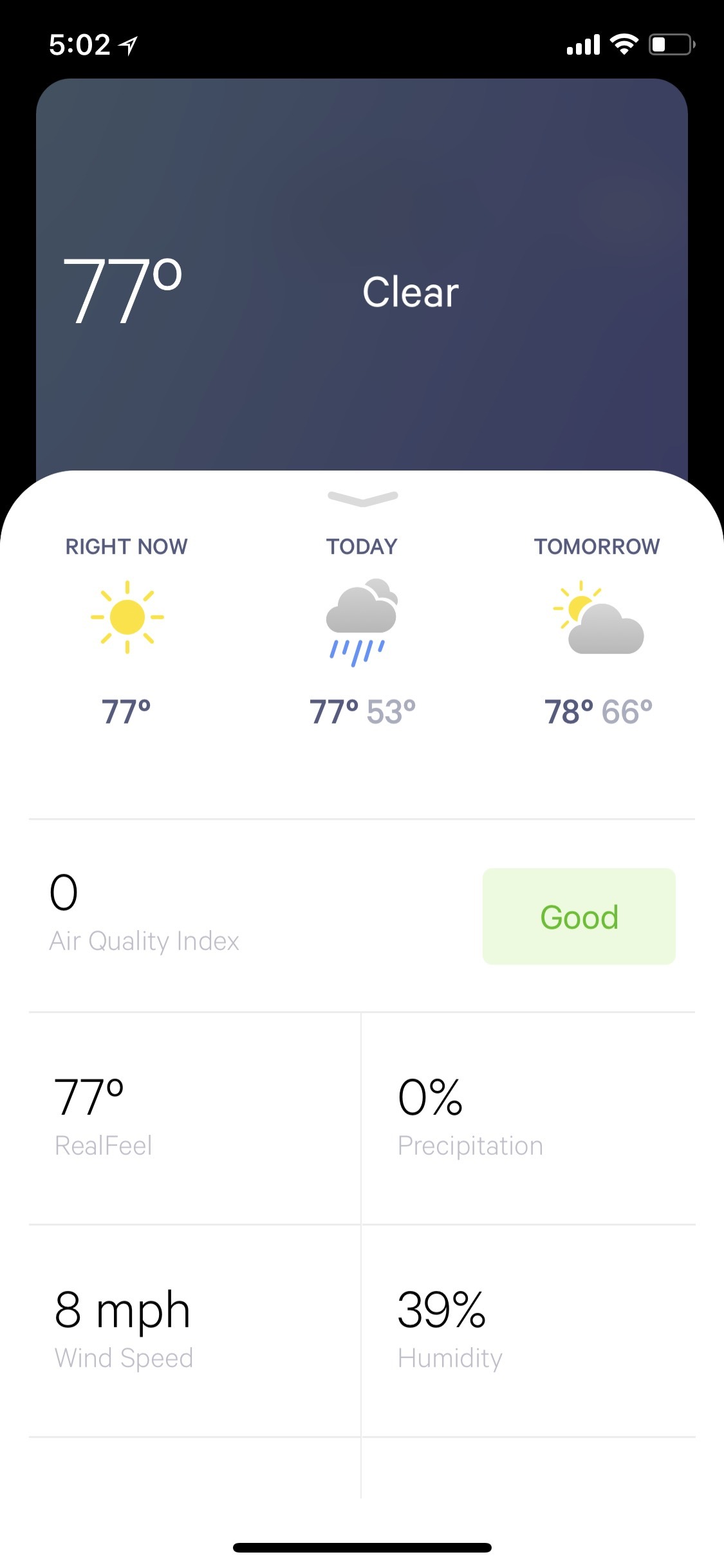The image displays a rectangular screenshot taken on a mobile device. At the very top, the black status bar includes the icons and text showing "502," "Location Services," four bars of data signal strength, full Wi-Fi signal, and less than half battery life.

Directly below the status bar, the screen transitions to a dark blue area indicating the current weather conditions: "77°F" with a "Clear" label. 

Prominently in the center is a pop-up menu with a white background, presenting detailed weather information. At the top of the menu, it reads "Across" followed by "Right Now," with a sun icon adjacent to the present temperature of "77°F." 

Further along in the pop-up menu, the forecast for "Today" is depicted with a cloud and rain icon, alongside temperatures of "77°F / 53°F." Next to it, "Tomorrow" forecasts a partly cloudy day, illustrated with a sun behind a cloud icon, and temperatures of "78°F / 66°F."

Beneath these headings, additional environmental data is provided: an "Air Quality Index" of "Zero," labeled as "Good" and highlighted in green. 

Following this, the menu indicates a "Real Feel" temperature of "77°F," with "0% Precipitation." Further information includes an "8 mph wind speed," "39% Humidity," and a thin horizontal black line spanning the center width of the screen. 

At the very top center of the pop-up menu, there is a small arrow icon pointing upwards, suggesting it can be tapped to collapse the menu. All descriptions within the menu are presented in light gray text for readability.